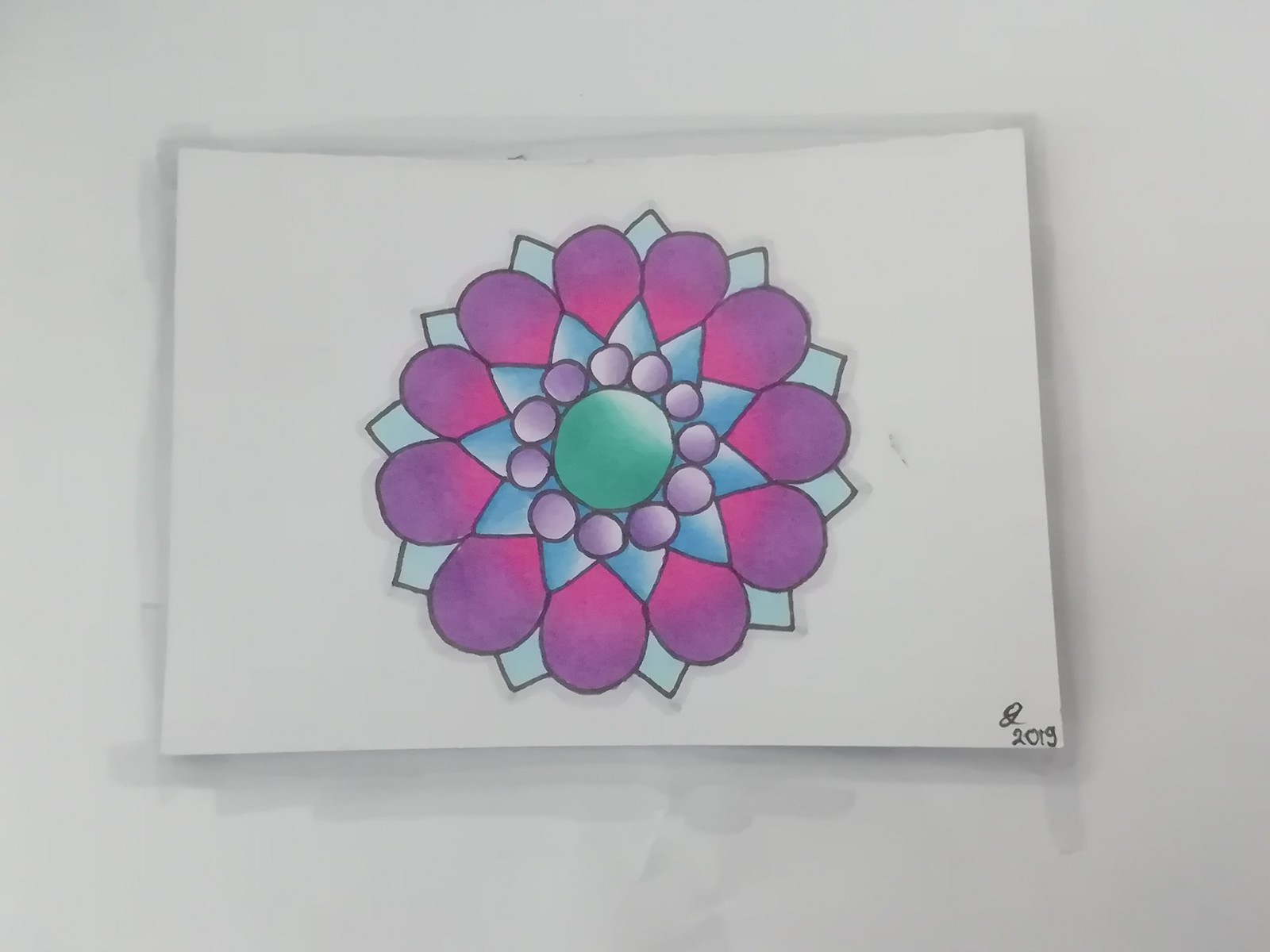The photograph showcases a detailed drawing on a white piece of paper, reminiscent of a mandala or a spirograph design. At the center of the image is a green circle, which is surrounded by a ring of smaller, light purple circles. Radiating out from this central arrangement are light blue triangles that create a star-like formation. Between each of these triangles, there are bright pink to purple petal shapes. Further accentuating the geometric pattern, additional light blue triangular shapes emerge between the petals. The entirety of the design is framed by a final row of outward-pointing triangles, maintaining the light blue hue. The lines and borders of these shapes are finely detailed, likely drawn with a felt pen. In the bottom right corner of the piece, there is a black squiggle resembling the initials of the artist, along with the inscription "2019." The intricate, repetitive nature of the drawing, combined with the vivid use of color, lends it a mesmerizing and almost floral aesthetic.